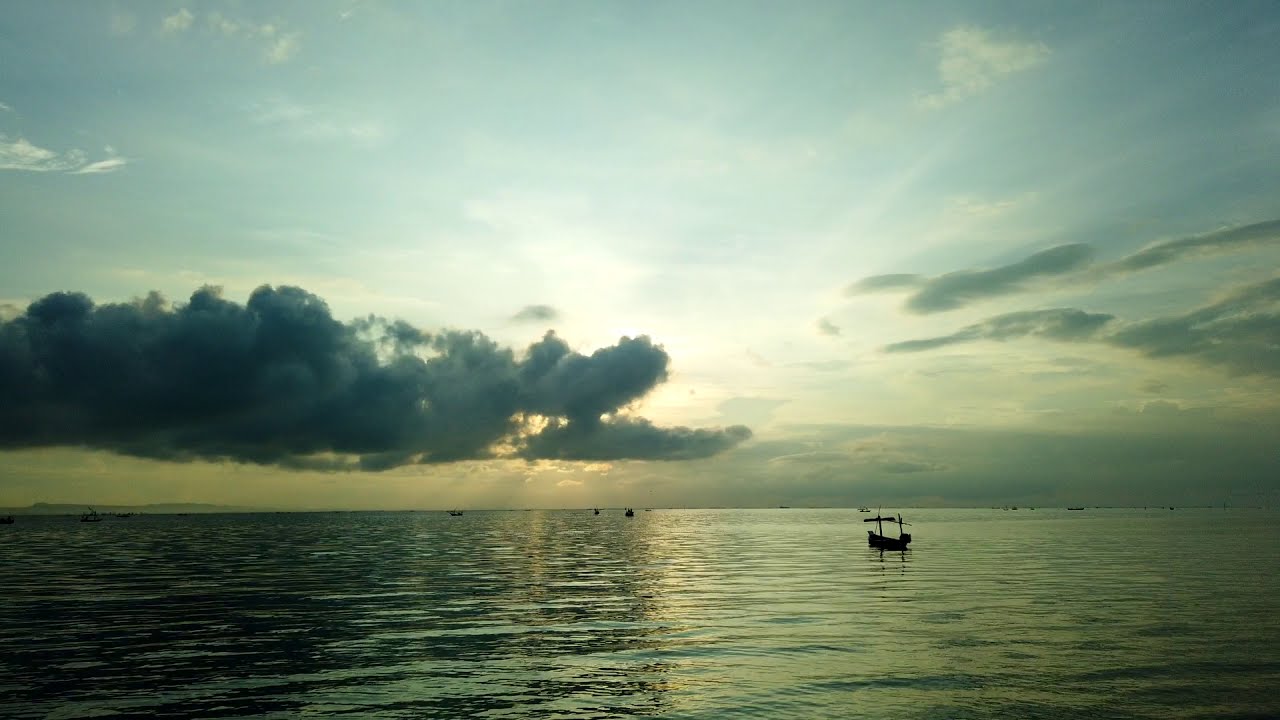The image captures a tranquil sunset over a body of water that occupies the bottom third of the frame. The water is dark, reflecting the sky's colors, with light ripples creating a shiny effect. To the left, a large, dark gray cloud casts a shadow on the water, which is noticeably darker beneath this cloud. The right side of the water glows with a lighter reflection. Small, dark-colored boats, including a brown sailboat with an upright mast but no sail, dot the surface, appearing as black spots in the distance.

The sky transitions from a deep blue at the top to a golden hue near the horizon, with gold-colored clouds clustering just above the waterline. A sun, partially obscured by clouds, shines through the center of the scene, casting a yellow glow. To the left, a thick, dark cloud dominates, slightly revealing patches of blue sky and wispy, hazy clouds. Meanwhile, the right side features scattered, darker clouds. Off in the horizon, faint traces of land with gentle elevation can be discerned.